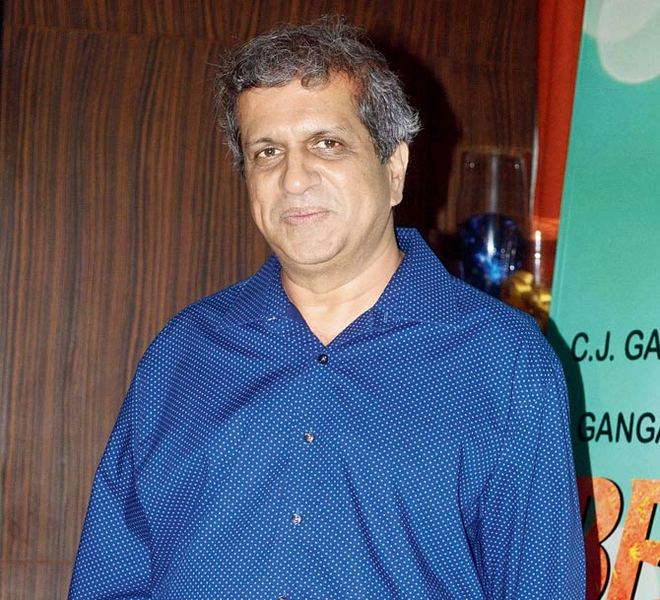This photograph captures an elderly man, possibly of Indian or Middle Eastern descent, standing casually with a faint smile directed at the camera. His dark hair peppered with white flecks showcases his aging. He dons a blue polka-dotted button-up shirt with its collar lying flat and the top button left undone, revealing a relaxed demeanor. The man, light-skinned with dark brown eyes and thin eyebrows, stands before a background of wooden paneling and various flags. One prominent flag is green and bears the partially visible text "CJ GA" and "gang" with some letters obscured, possibly hinting at an event or a lecture. Beside him, on a shelf, sit a few glasses, while a glass container holding a lit blue candle and another candle amongst gold embroidery are also visible. A red pillar with a blue sign, accentuated with white circles, further decorates the scene, adding a sense of ceremonial or formal ambiance.